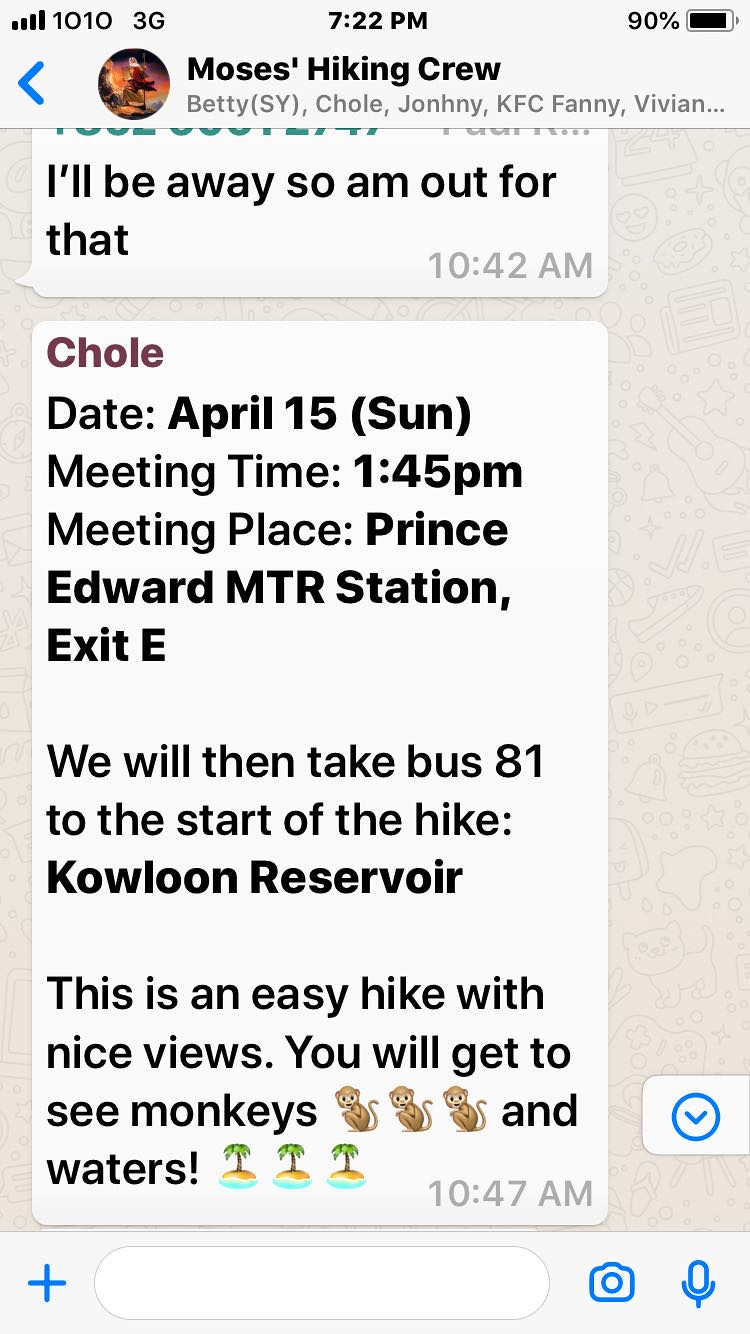The image is a detailed screenshot of a messaging app on a mobile phone, displaying a conversation within a group chat titled "Moses Hiking Crew." At the top of the screen, a circle with a picture is visible, alongside text indicating battery life at 90%. The first message, timestamped at 10:42 a.m., reads, "I'll be away so I'm out for that." Below this, a message from Chloe states, "Date: April 15th, Sunday. Meeting time: 1:45 p.m. Meeting place: Prince Edward MTR Station, Exit E. We will then take bus 81 to the start of the hike, Kowloon Reservoir. This is an easy hike with nice views. You will get to see monkeys and waters." The screenshot occupies the entire image, making additional objects or background details unnecessary. The color scheme includes tan, black, blue, orange, yellow, green, and purple. The bottom of the screen shows a search bar and three icons, emphasizing the mobile interface.